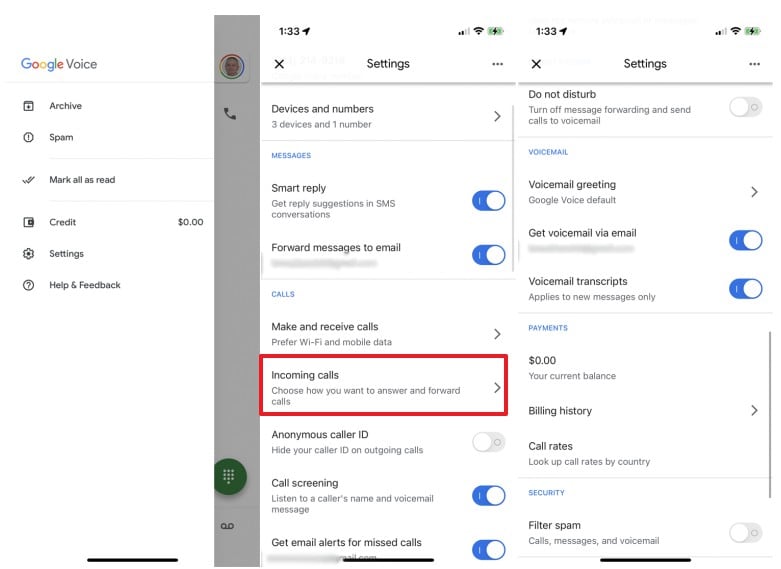The image features a screenshot of a smartphone's settings menu, specifically focusing on communication settings. The section highlights various features related to devices and notifications. It mentions three main devices and one associated number. Here's a detailed breakdown:

- **Messages**: Includes options for enabling Smart Replies for SMS conversations, as well as settings to forward messages to email.
- **Calls**: Allows making and receiving calls, with preferences for using Wi-Fi and mobile data. It includes options for handling incoming calls, choosing how to answer and forward them. Notably, the "Incoming Calls" section and subsequent settings are enclosed in a red box.
- **Caller ID**: Features settings for an anonymous caller ID, enabling the hiding of your caller ID on outgoing calls.
- **Call Screening**: Provides options to listen to a caller's name and voicemail message, along with receiving email alerts for missed calls.
- **Do Not Disturb**: Allows turning off message forwarding and sending calls directly to voicemail.
- **Voicemail**: Includes settings for customizing voicemail greetings with Google's default options, receiving voicemail via email, and applying voicemail transcripts to new messages only.

This comprehensive and detailed caption delineates each available setting for effective management of communication functionalities on the device.